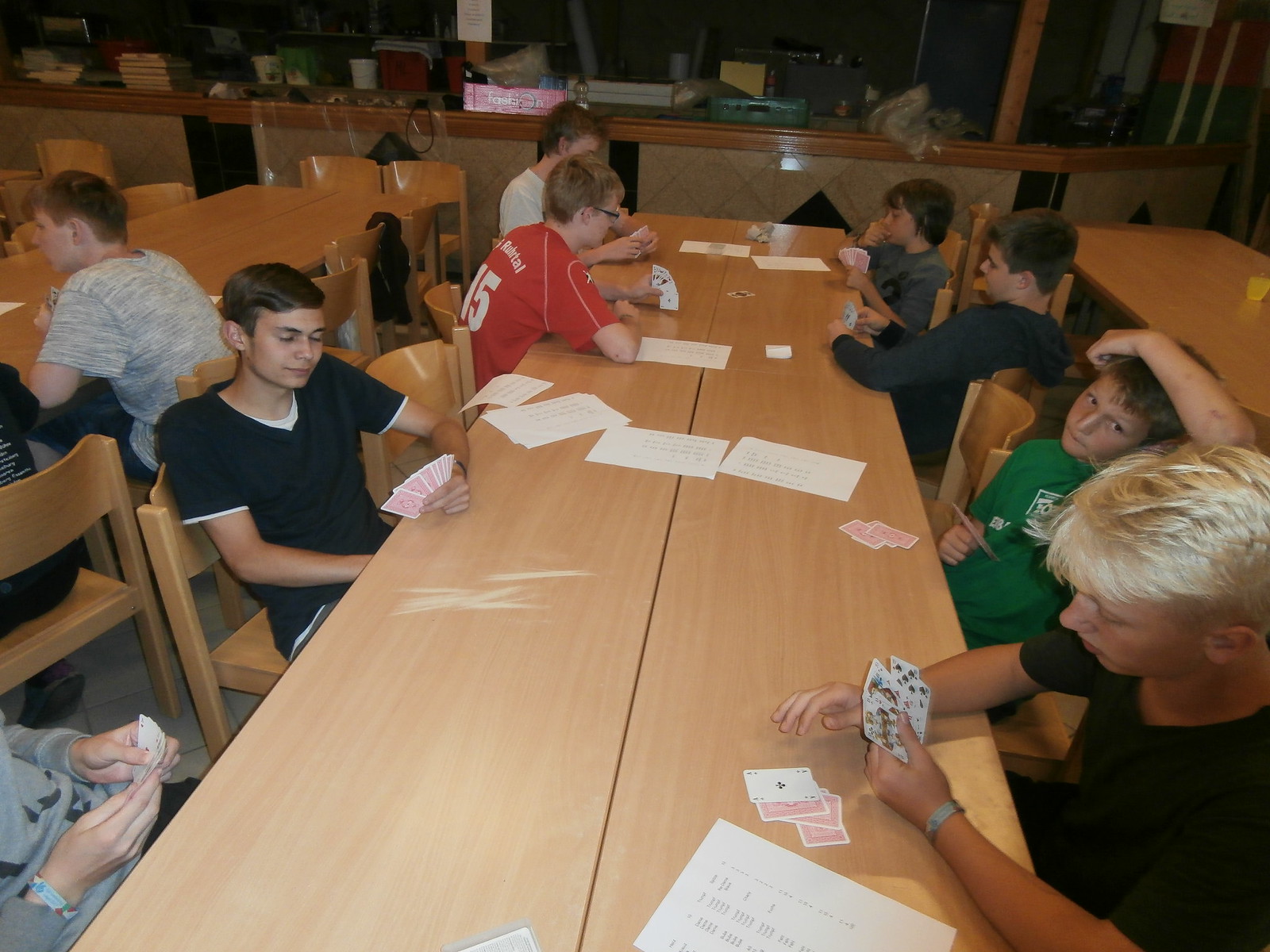In a bustling cafeteria setting, three long wooden tables dominate the foreground, each populated by groups of young boys engaged in an animated card game. The tables are arranged in a parallel configuration, with each one accommodating several players. On the table closest to the viewer, four boys are seated on one side and three on the opposite side, all deeply focused on the cards in their hands. Behind this main group, another table seats four boys on one side and two on the other, similarly absorbed in their game.

Scattered haphazardly across the tables are various papers, the contents of which are unclear, adding to the casual, impromptu atmosphere of the gathering. In the background, a counter indicative of a cafeteria-style arrangement is visible, further grounding the setting in what appears to be a school dining area. The boys, who range in age from junior high to early high school, are dressed in a variety of shirts: some green, some black, one white, one red, and one gray.

The scene is a lively tableau of youthful camaraderie and leisure, capturing a moment of shared enjoyment amidst the everyday routine of school life.